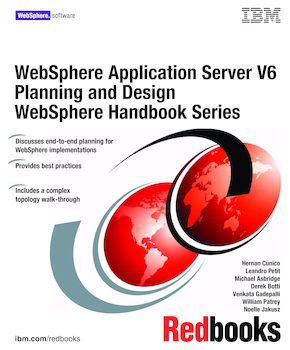The image is likely a cover for a book or an instructional manual related to IBM's WebSphere software. Dominating the top right of the cover is the IBM logo. Centrally, the text reads, "WebSphere Application Server v6, Planning and Design WebSphere Handbook Series," all in black. This main title is followed by additional descriptive text which states, "Discusses end-to-end planning for WebSphere implementations, provides best practices, includes a complex topology walkthrough." Below this, multiple authors' names are listed on the right side. The central graphic feature of this cover includes two red-toned globes with shading: one displaying Africa, Asia, and Australia, and the other showing North and South America, effectively depicting both sides of the world. At the bottom left, there is a web address that reads "ibm.com/redbooks." Additionally, the title "redbooks" appears at the bottom, with 'red' in red text and 'books' in black text.